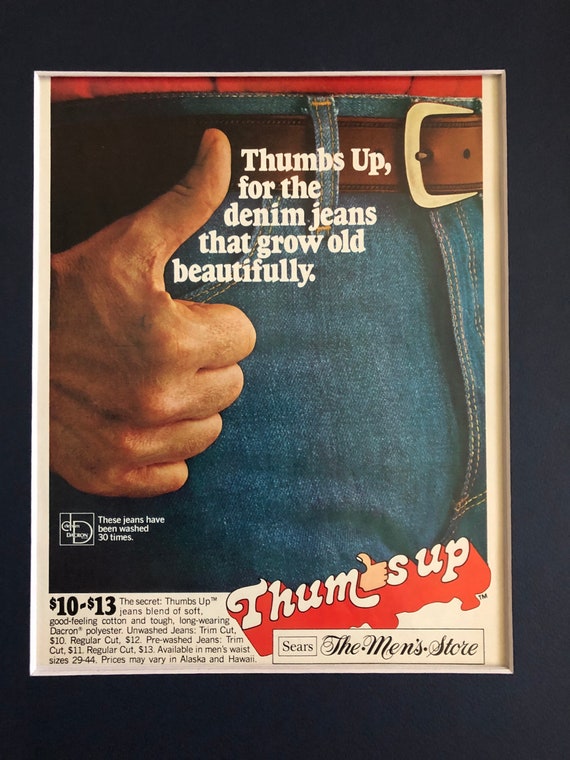The rectangular advertisement poster features a close-up view of a pair of dark blue denim jeans, accented by a brown leather belt with a gold buckle. The jeans are worn by a person of Caucasian descent with tan skin, who is giving a thumbs-up gesture with their right hand. A small portion of a red shirt is visible, tucked into the jeans.

The background of the poster is a flat black with a white border delineating the ad space. Central to the design, in bold white letters beside the thumb, is the tagline: "Thumbs up for the denim jeans that grow old beautifully." A square logo featuring a small 'd' and a capital 'D' indicates the jeans have been washed 30 times.

At the bottom right of the poster, there is a red background with animated thumbs-up icon and the text "Thumbs up." Adjacent to it, the Sears logo and the phrase "the men's store" are displayed in a white rectangle.

The pricing details on the poster read: "Ten to thirteen dollars. The secret thumbs up jeans blend of soft, good-feeling cotton and tough, long-wearing Dacron polyester. Unwashed jeans: Trim cut, $10; Regular cut, $12. Pre-washed jeans: Trim cut, $11; Regular cut, $13." Men's waist sizes range from 29 to 44, with a note that prices may vary in Alaska and Hawaii.